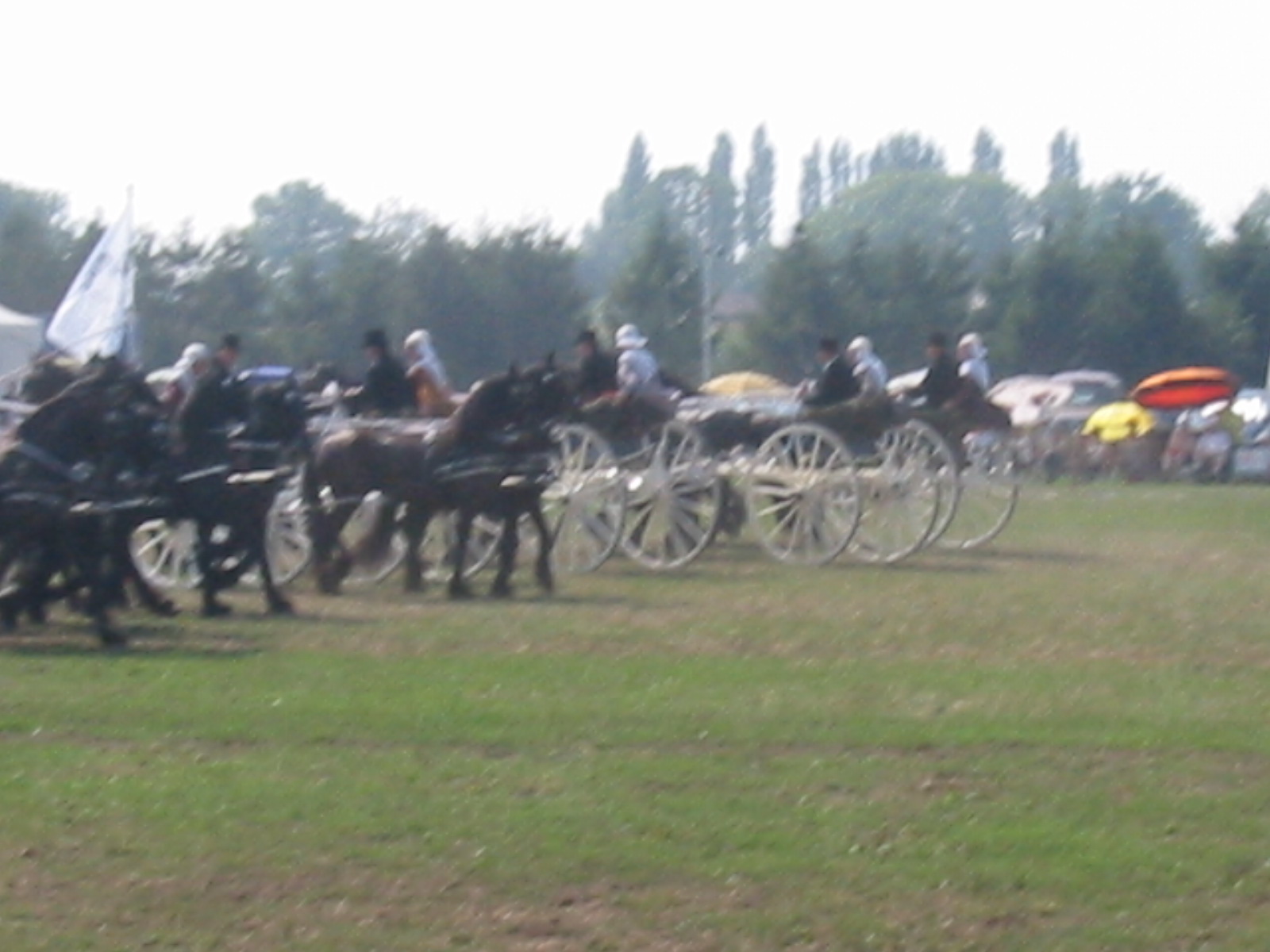The photograph appears to capture a historic reenactment or a staged event featuring horse-drawn carriages on a grassy field. Despite its blurriness, several details are discernible. The field is a mix of light green and brown grass, and the background features a vivid array of dark green trees beneath a sky that blends from bright gray to cloud-strewn white. To the left, a white flag stands prominently. 

In the foreground and slightly to the right, pairs of brown horses are harnessed to carriages with white wheels and spokes, their straps visible around their chests. The drivers, dressed in black coats and top hats, share their seats with individuals in silver outfits. 

Among the spectators are people seated beneath a medley of umbrellas in orange, yellow, and white hues, while others mill about a possible nearby parking area. Notably, women dressed in blue dresses with white caps and men in black coats mingle amidst the scene, adding to the historic ambiance. The evocative tableau is a picturesque blend of somber and festive, unified by meticulous details that suggest a well-coordinated gathering or depiction of days gone by.